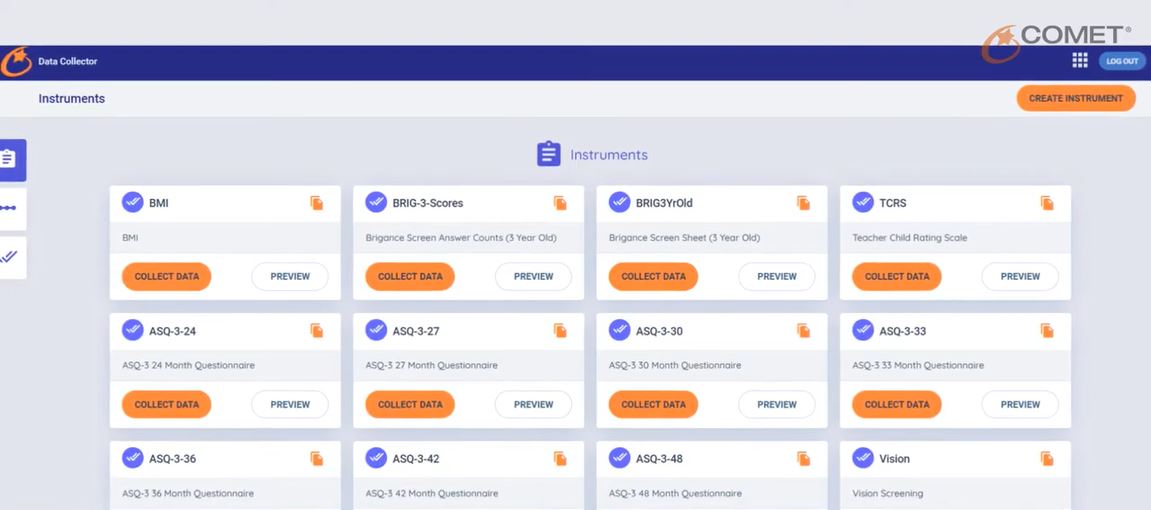This screenshot from Comet's Data Collector interface showcases a structured and organized layout of data collection instruments. The main display is composed of three rows, each containing four uniform boxes. In total, there are twelve boxes. Each box features a consistent design, marked with a checkmark inside a blue circle, an orange oval labeled "Collect Data," and a white oval labeled "Preview." Additionally, an icon resembling a file cabinet is present in each box, suggesting the availability of various data categories.

In the upper right-hand corner, an orange oval button labeled "Create Instrument" is prominently displayed. This button indicates the user’s ability to create new data collection instruments.

The specific data collection instruments are organized as follows:
- **First Row:** BMI, BRIG-3 Scores, BRIG-3Y (Old), and TCRS.
- **Second Row:** ASO-3-24, ASO-3-27, ASO-3-30, and ASO-3-33.
- **Third Row:** ASO-3-36, ASO-3-42, ASO-3-48, and Vision.

The consistent layout and labeling ensure that users can efficiently navigate and utilize the data collection features provided by Comet's Data Collector.